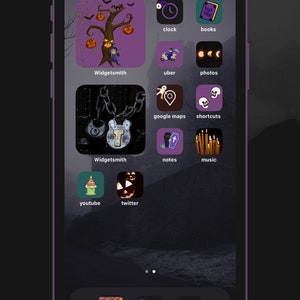This image showcases a mock-up of an iPhone displaying a Halloween-themed icon pack. The iPhone, encased in a distinctive purple cover complete with matching buttons, reveals its vibrant display despite both the top and bottom portions of the photo being cropped out. Dominating the screen are large, Halloween-inspired icons, including a spooky tree with pumpkins and metal chains dangling from its branches. Other prominent icons depict a pumpkin, a coffin, candles, and skulls. The backdrop of the phone screen features a haunting, foggy, and deserted scene, perfectly complementing the eerie atmosphere. Notably, the background behind the entire phone mirrors this same spooky wallpaper, reinforcing the Halloween theme. This detailed image highlights a creative and cohesive Halloween cell phone theme or icon pack, designed to fully immerse users in the festive spirit.